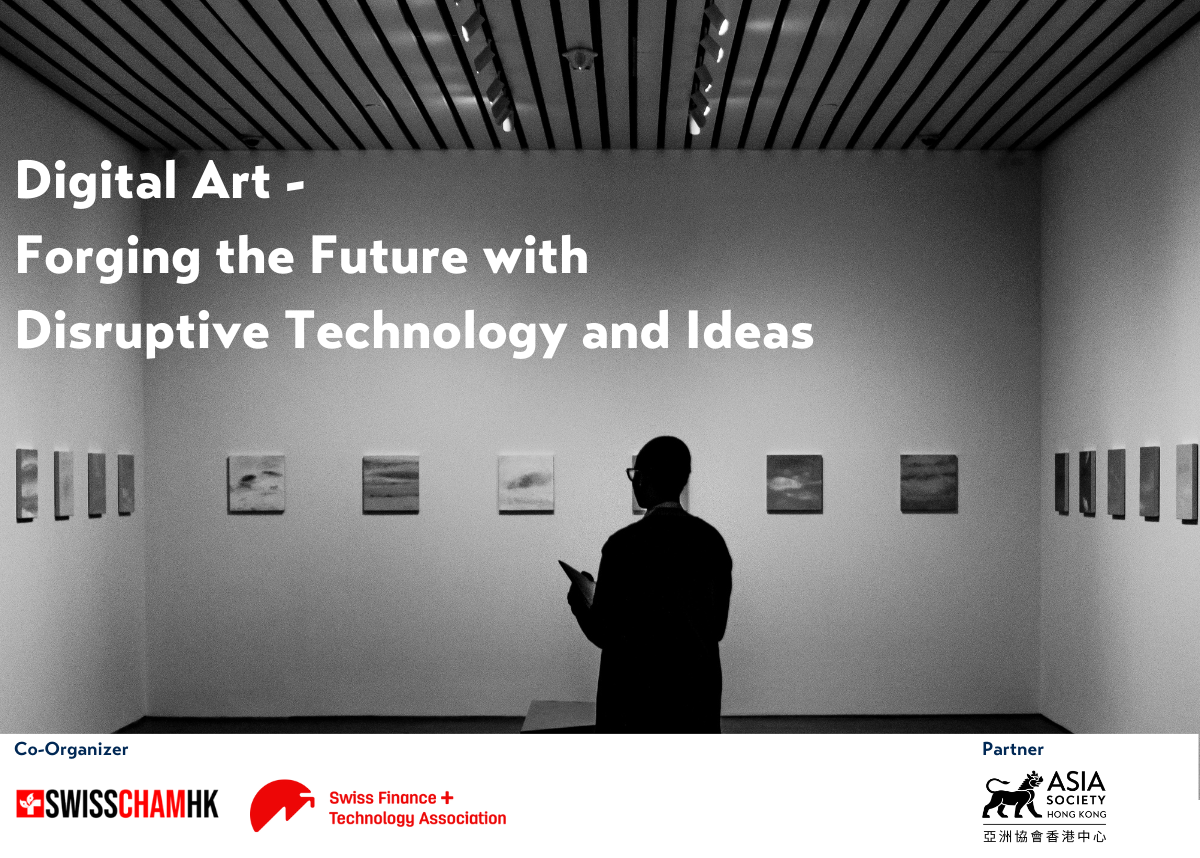The image is a poster featuring a black-and-white photograph of a bald or shaved-headed individual standing in the middle of a white-walled gallery. The gallery's walls are uniformly adorned with thirteen small, regularly spaced square canvases, primarily in shades of black and white. The ceiling features striped bars and lights that illuminate the artworks. In the upper left quadrant of the image, white text reads, "Digital Art – Forging the Future with Disruptive Technology and Ideas." Below the main image, on a white background, blue text in the bottom left corner states "Co-Organizer," accompanied by logos including "Swiss" in black, "Cham" in red, and "HK" in black, along with a white cross on a red background. To the right, in red text, is the logo of the "Swiss Finance Technology Association," depicted as a stylized half circle with a triangle. In the bottom right corner, blue text reads "Partner," above a black logo featuring a Chinese lion design and the text "Asia Society Hong Kong," with accompanying Chinese characters below a thin black line.